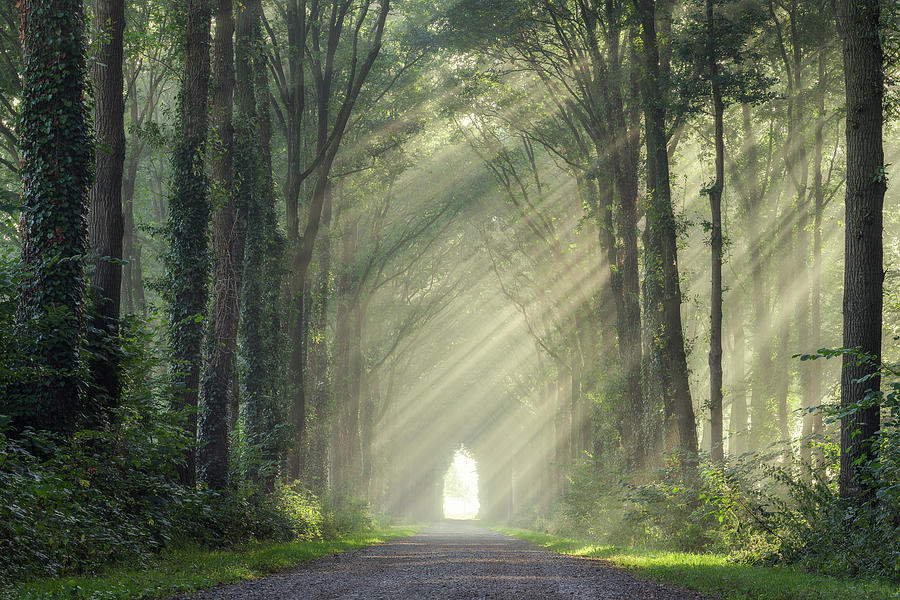The image depicts a picturesque landscape of a forested trail, where a wide gravel path stretches straight down the middle. On either side of the path lies a narrow strip of green grass, about the width of a riding lawnmower, along with patches of bushes. Tall trees with dark brown trunks and some adorned with dark green ivy line both sides of the trail, forming a lush tunnel-like canopy overhead. Sunbeams penetrate the foliage from the right side, casting diagonal beams of white light that illuminate the trail and create a peaceful, almost foggy atmosphere. At the end of the trail, a white archway floats in the distance, adding to the enchanting tunnel effect created by the interlacing branches and leaves above.